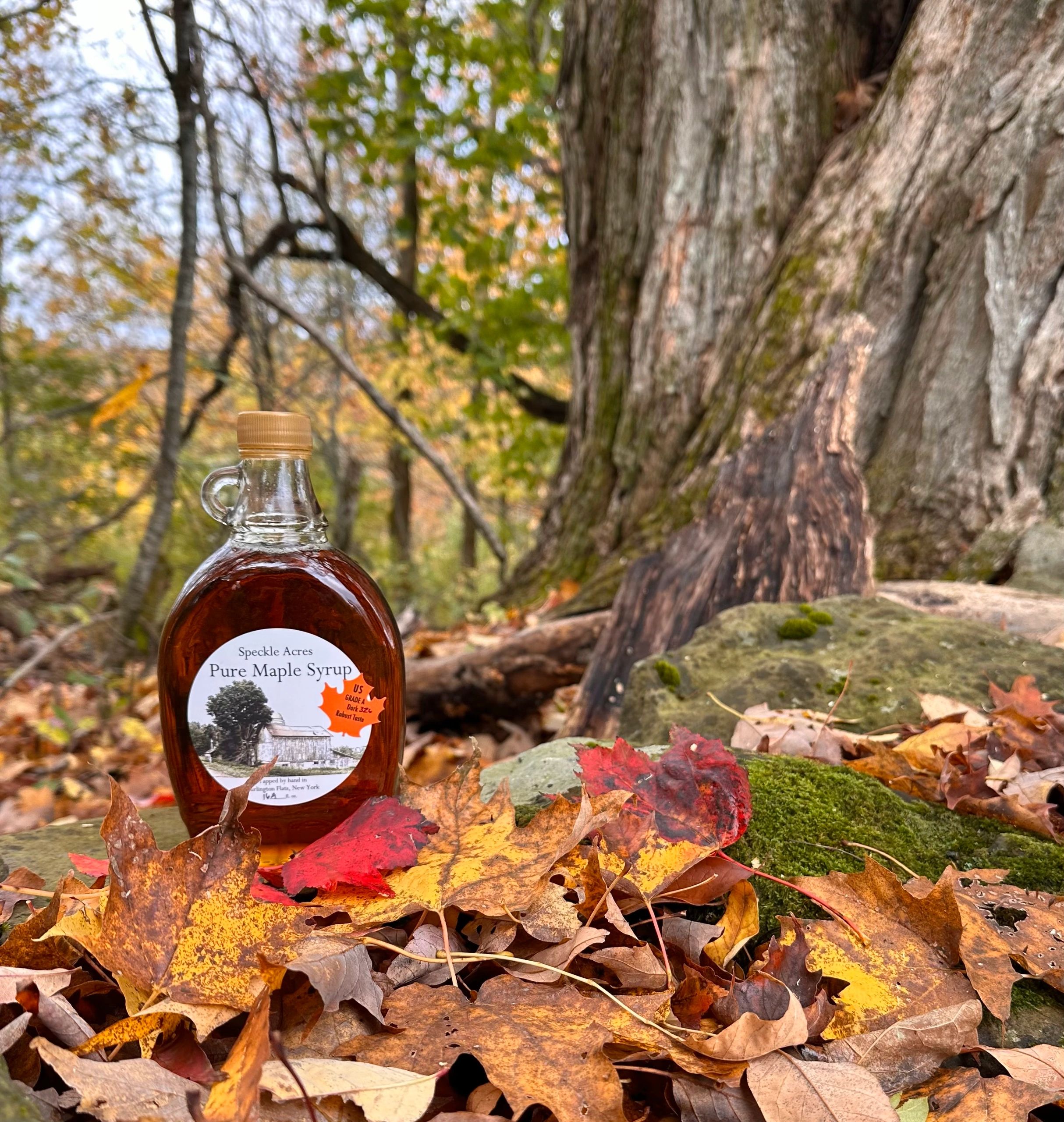In a serene forest setting, a thick tree stump, covered in green moss, stands amidst fallen maple leaves in vibrant hues of red, orange, yellow, and brown. A glass bottle of 'Speckle Acres Pure Maple Syrup,' adorned with a white label featuring an orange maple leaf and an illustration of a tree and barn, rests atop the colorful leaves. The bottle, capped with a tan lid and equipped with a small handle, exudes rustic charm. Behind the syrup bottle, the scenery extends to smaller trees with green and yellow leaves, against a backdrop of blurred foliage, blue sky, and sunlight filtering through the branches, adding a touch of warmth to the autumnal tableau.